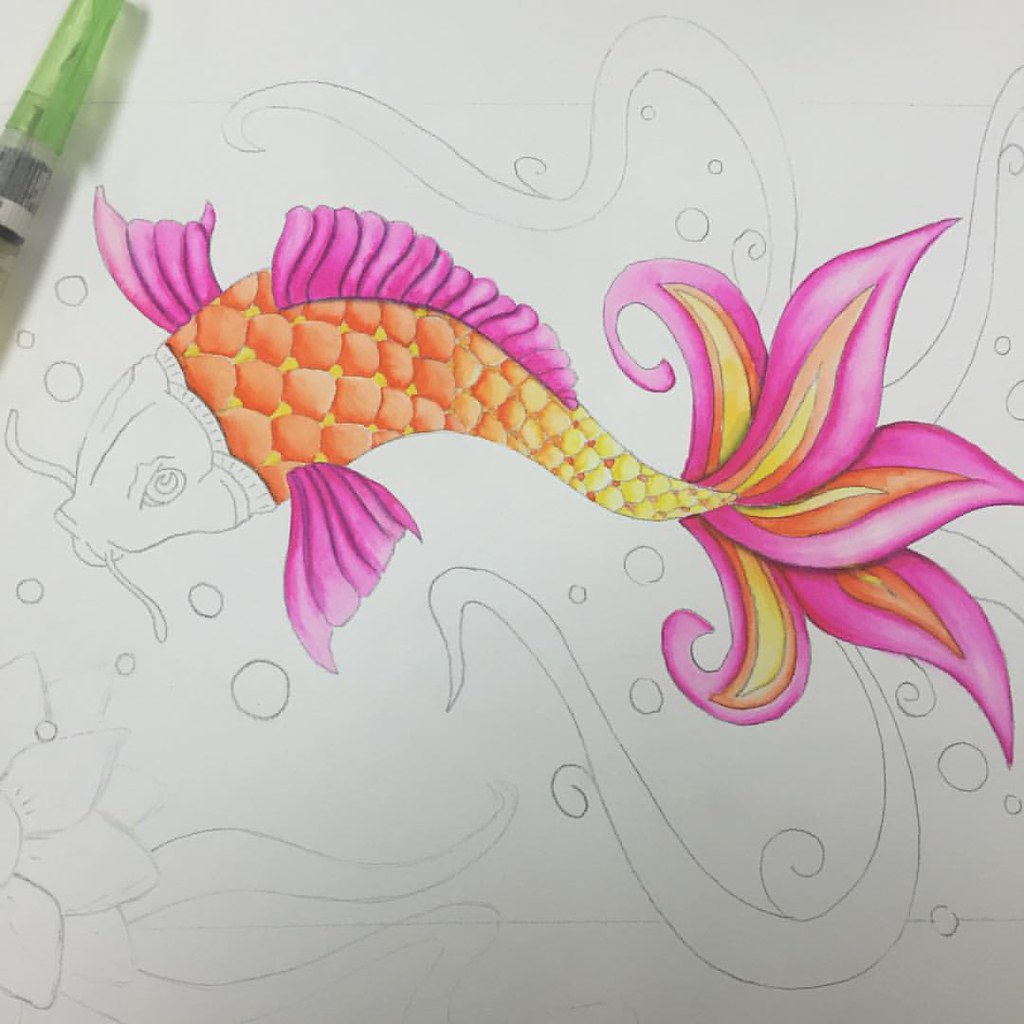In this photograph taken from an above view, we see a vibrant hand-drawn depiction of a stylized fish on whitish paper. The fish, which resembles a catfish or a fighter fish, features an intricate and colorful design. Its body is adorned with orange scales transitioning to pink towards the fins. The fins—left, right, and top—are colored pink, while the elaborate tail fans out into five petal-like flaps, each with tips in shades of pink, yellow, and orange. The head of the fish, sporting characteristic catfish whiskers, remains uncolored, sketched only in grey pencil lines.

Surrounding the fish are artistic bubbles and stylized swirling water patterns, also rendered in grey pencil, suggesting an underwater scene. Visible in the top left corner of the artwork is the tip of a pencil with a translucent green lid, hinting that the image is a work in progress. Additionally, there appears to be an indistinct shape, possibly a jellyfish or an underwater flower, rendered in pencil and moving in the same direction as the fish, enhancing the aquatic theme of this partially colored, intricate drawing.